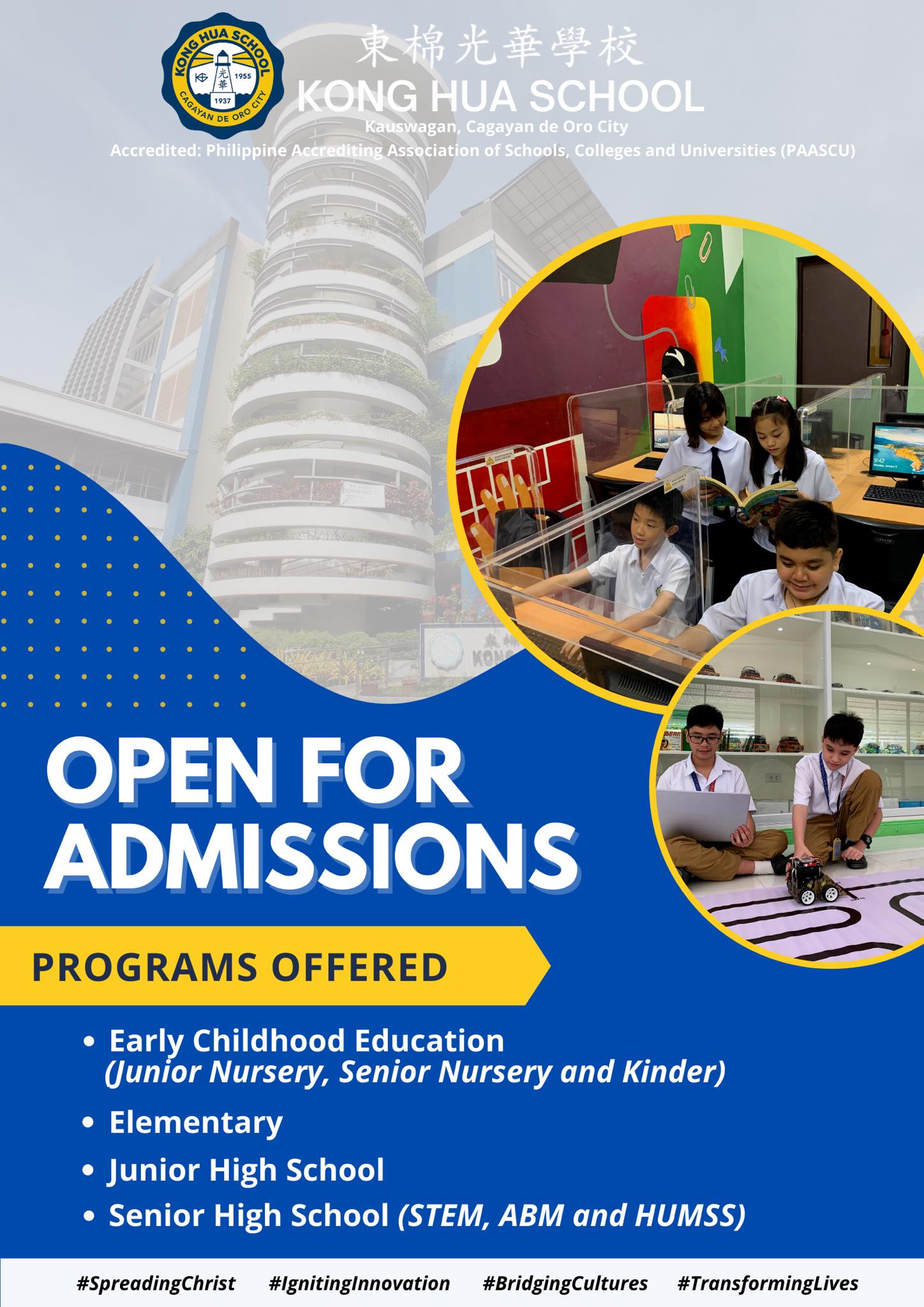This image is a screenshot of an online advertisement for Kong Hua School. At the top, there are Chinese characters, followed by the English text "Kong Hua School." To the left of this text is the school's seal: a yellow circle encompassing the words "Kong Hua School," with a white lighthouse at the center. Two yellow beams emanate from the top left and right of the lighthouse. Additionally, there is blue text that reads "Kagayan de Oro City."

Below the name "Kong Hua School," more text states, "Kagayan de Oro City, accredited by the Philippine Accrediting Association of Schools, Colleges, and Universities (PAASCU)." 

In the background, a filtered and slightly blurry image of the school's premises can be seen, including a prominent lighthouse-like tower.

Superimposed over the background is a yellow circle featuring a photograph of young Filipino children studying in clear plastic-separated cubicles. The entire scene conveys an educational and organized environment.